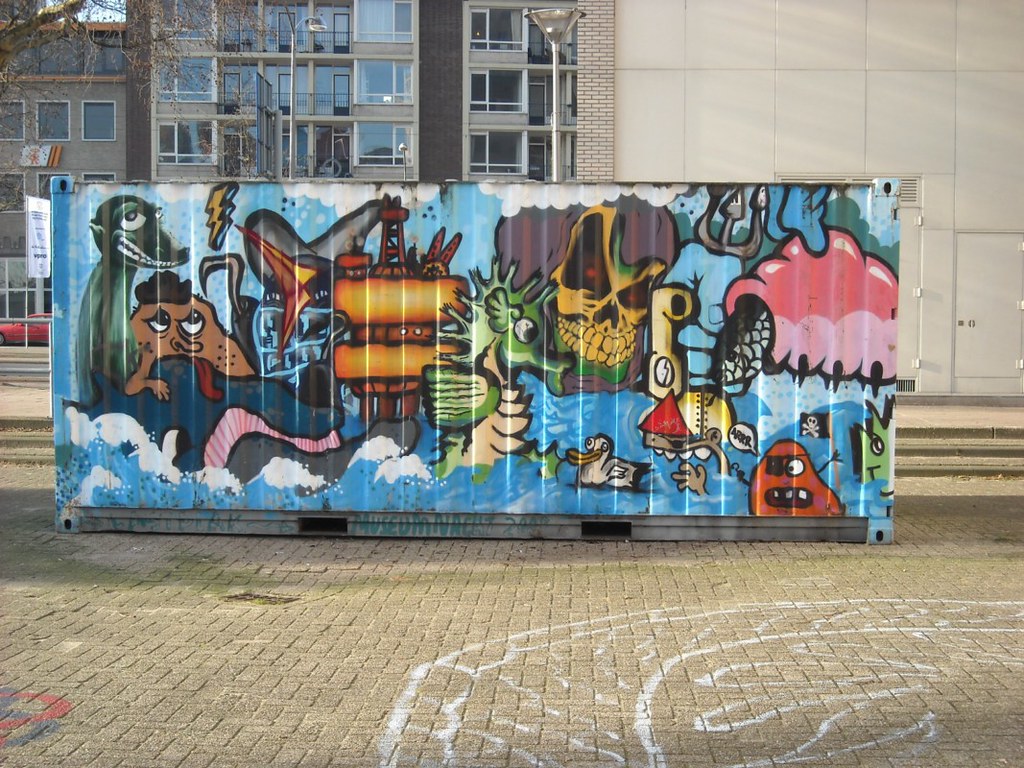The photograph captures an urban courtyard with a tan brick surface, framed by apartment buildings and a blank wall in the background, alongside a street lamp. Central to the image is a large metal surface, likely a dumpster, adorned with a vivid, graffiti-style mural. The mural features a fantastical underwater scene with an array of colorful, cartoon-like sea creatures, including a recognizable duck and a stylized seahorse, amidst anemones and abstract shapes. Dominating the scene are a giant skull face and what appears to be an oil derrick. The mural's palette spans purple, orange, blue, green, yellow, pink, red, and black. In front of the mural, there's a chalk drawing on the gray brick street, adding another layer of artistic expression to the setting, which also includes a visible car and a street lamp in the background.